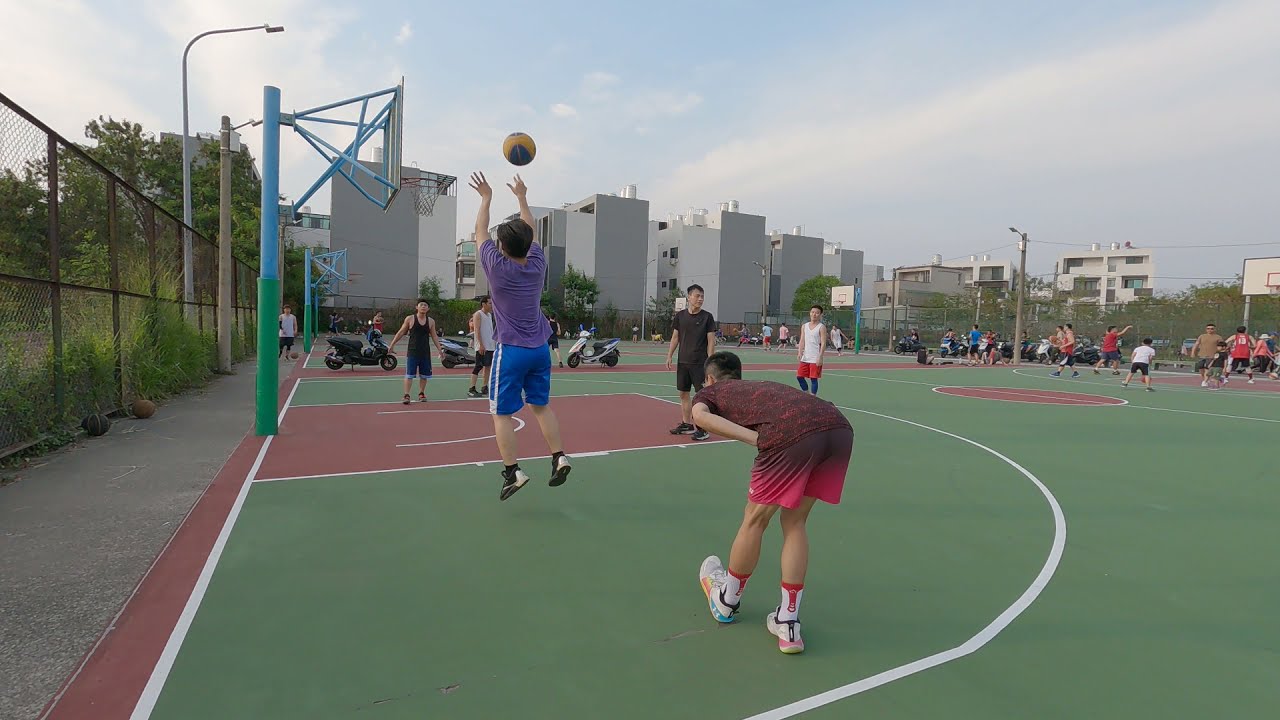The image depicts a vibrant outdoor sports facility featuring multiple basketball courts with a distinct red clay and green color scheme, outlined with white lines. The photo, taken from a corner of one court, captures a bustling cityscape with apartment complexes, small trees, and grassy areas visible beyond a somewhat rusty chain-link fence lining the courts. The sky forms a backdrop above the urban environment.

In the foreground, a young man wearing a purple shirt and blue shorts is in mid-air, executing a jump shot from just outside the key, which is colored red. Nearby, another young man in a red shirt and mismatched pink or red shorts is bent over near the three-point line, poised in anticipation. Several other young men are scattered across the courts, participating in two separate games happening on either side of the main court. One player in the distance, clad in a white shirt with red shorts, stands outside the white lines of the court.

A side view of a basketball net is visible towards the left middle of the image, with onlookers and participants positioned strategically to rebound the ball. Additional courts in the background are similarly active, with groups of players engaged in their own games. Motorcycles are also lined up in the space between the courts. The presence of lights suggests that the facility is equipped for nighttime play.